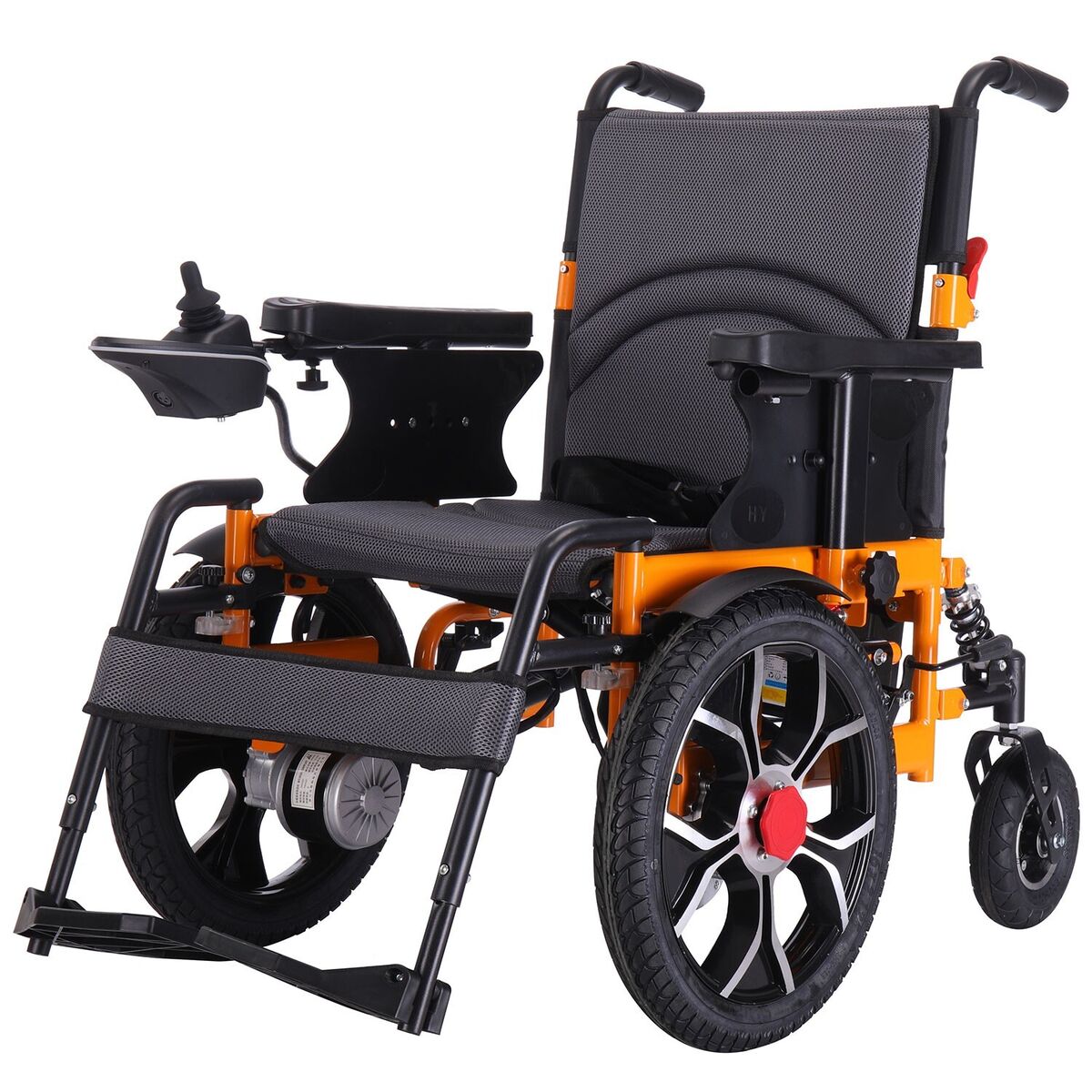The image showcases a sleek, modern wheelchair in a slightly slanted position, offering a clear view of its sophisticated design. The majority of the wheelchair's frame is predominantly black, complemented by a black-gray mesh seat that promises comfort and support. Notably, this wheelchair appears to be motorized, identifiable by a visible joystick control on the right-hand side, which allows for effortless maneuverability. The black frame is accentuated with striking orange details, particularly on the metal components connecting the wheels. The wheelchair features a large wheel at the back and a smaller, yet significant, wheel at the front to ensure stability and smooth transportation. While the left side of the wheelchair remains partially obscured, it is presumable that it mirrors the intricate design and features observable on the right.